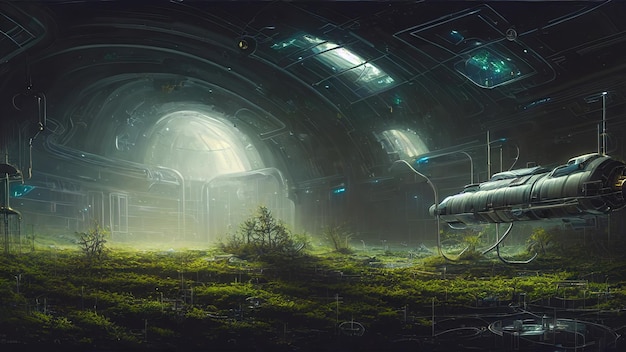The image depicts a beautifully rendered sci-fi drawing that showcases the inside of a metal-domed, subterranean room or spaceship interior. The ceiling curves overhead and features multiple openings that allow beams of sunlight to penetrate the otherwise dimly lit space. Numerous pipes and wires run along the curved ceiling, adding to the sci-fi aesthetic. The far end of the room is brightly illuminated, suggesting a strong light source from the ceiling above. 

The ground is covered with dirt, thriving green grasses, and small, growing trees, creating an unexpected garden-like environment within this metallic room. Water appears to be dripping inside, likely from a series of sprinklers or watering systems integrated into the structure. On the right side of the image, there is a low, cylindrical metal object that could be a spaceship or a specialized farming machine, distinguished by its squat shape and elevated stance on metal supports. This fusion of nature and advanced technology creates a striking and intricate visual experience.